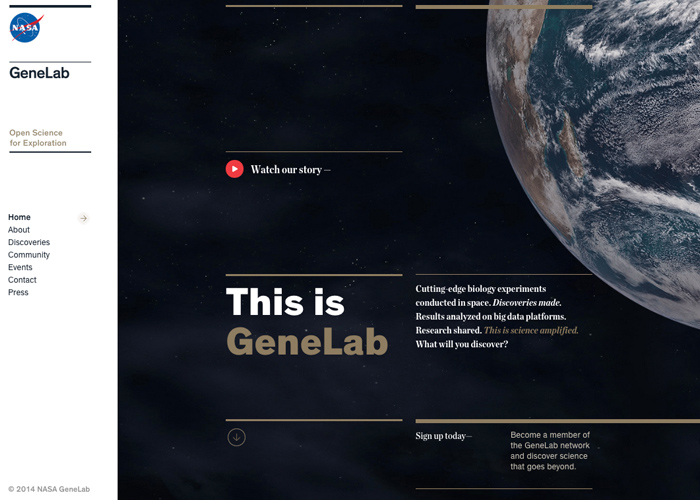This detailed caption describes a cropped screenshot of the NASA GeneLab webpage with clear and precise information about its layout and design elements.

---

**Description of NASA GeneLab Webpage Screenshot**

The cropped screenshot showcases the NASA GeneLab webpage with a layout rich in visual elements and organizational features. 

1. **Top Left Area:**
   - **White Banner**: Dominated by the NASA logo prominently placed at the top left corner.
   - **Black Bar**: Directly below the banner, a thin black bar displays the word "GeneLab" in large black letters.

2. **Tagline:**
   - Underneath the black bar, the phrase "Open Science for Exploration" is displayed in light gray letters.

3. **Left Sidebar:**
   - **Vertical Column of Categories**: A vertical menu lists categories such as Home, About, Discoveries, Community, Events, Contact, and Press. The "Home" category is highlighted as selected.

4. **Main Content (Right Side):**
   - **Earth Image**: A striking, large photograph of Earth positioned toward the top right corner blends into the vastness of outer space.
   - **Central Elements**: 
     - A thin gold bar is positioned towards the center.
     - Below this bar, a red YouTube play button invites users to "Watch Our Story" in small white letters.
     - Another thicker gold bar below contains the text "This is GeneLab" with "GeneLab" written in very large tan-ish gold letters.

5. **Description Section:**
   - Adjacent to "This is GeneLab", another thin gold bar sits above a description of the website.

6. **Bottom Left Area:**
   - **Gold Bar and Circle**: A gold bar sits above a gold circle featuring a downward-pointing gold arrow.
   - **Sign-Up Information**: To the right of this circle, a thick gold bar with small white letters encourages users to "Sign Up Today", followed by information on how to become a member.

This detailed description offers a comprehensive overview of the key elements and layout of the NASA GeneLab webpage as depicted in the cropped screenshot.